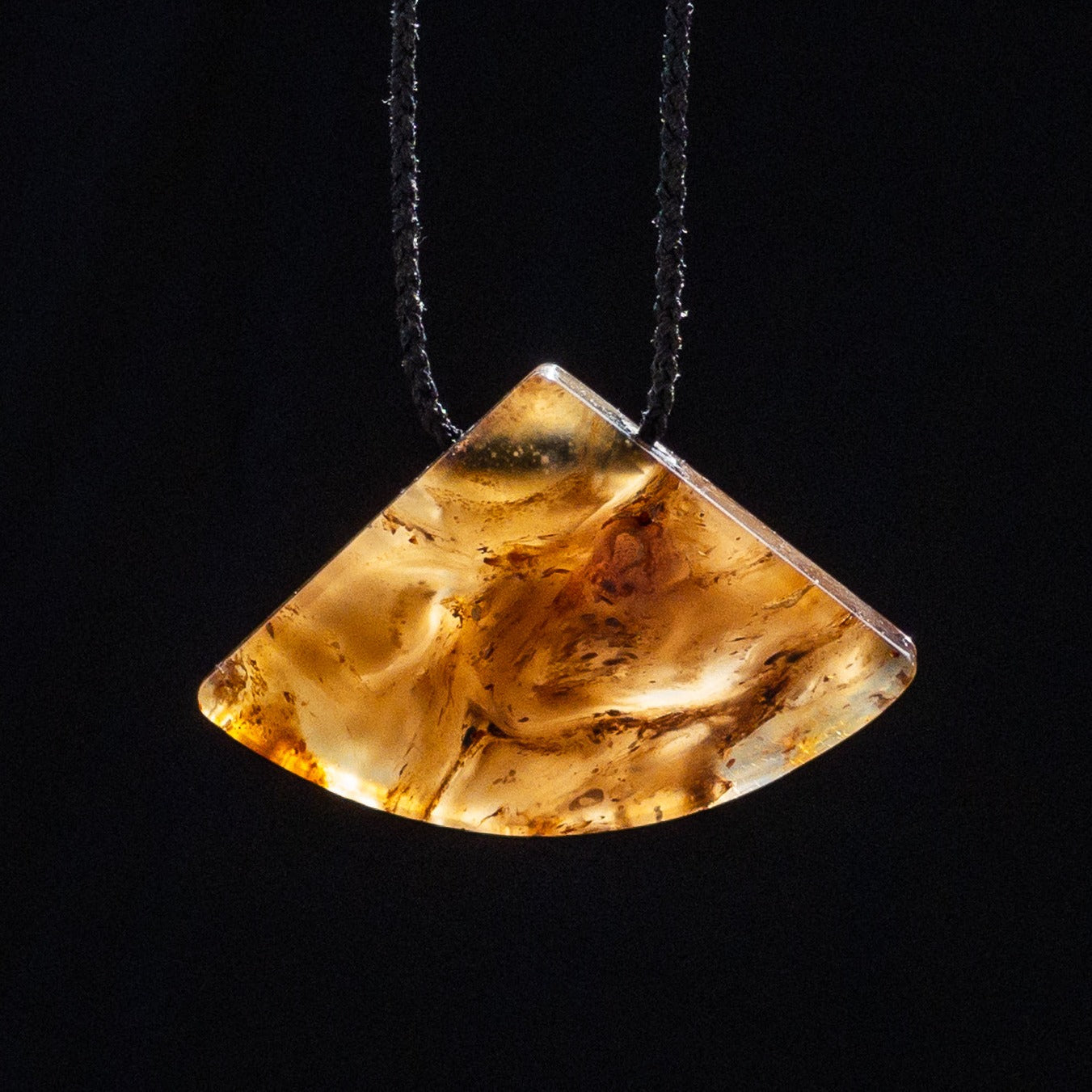This image features a close-up view of a pendant against a black background. The pendant is suspended from a black, braided string or twine, which enters the frame from the top, split into two strands. The ropes thread through two holes situated near the pointed top of the pendant, which exhibits a unique geometric design resembling a folded cone or a curved triangle. The pendant showcases a mix of colors, predominantly brown, with additional splotches of black, light yellow, dark brown, and hints of white. Its texture appears wooden or marble-like, adding an intricate visual depth to the piece. The background's stark blackness highlights the pendant’s detailed and multi-toned surface.